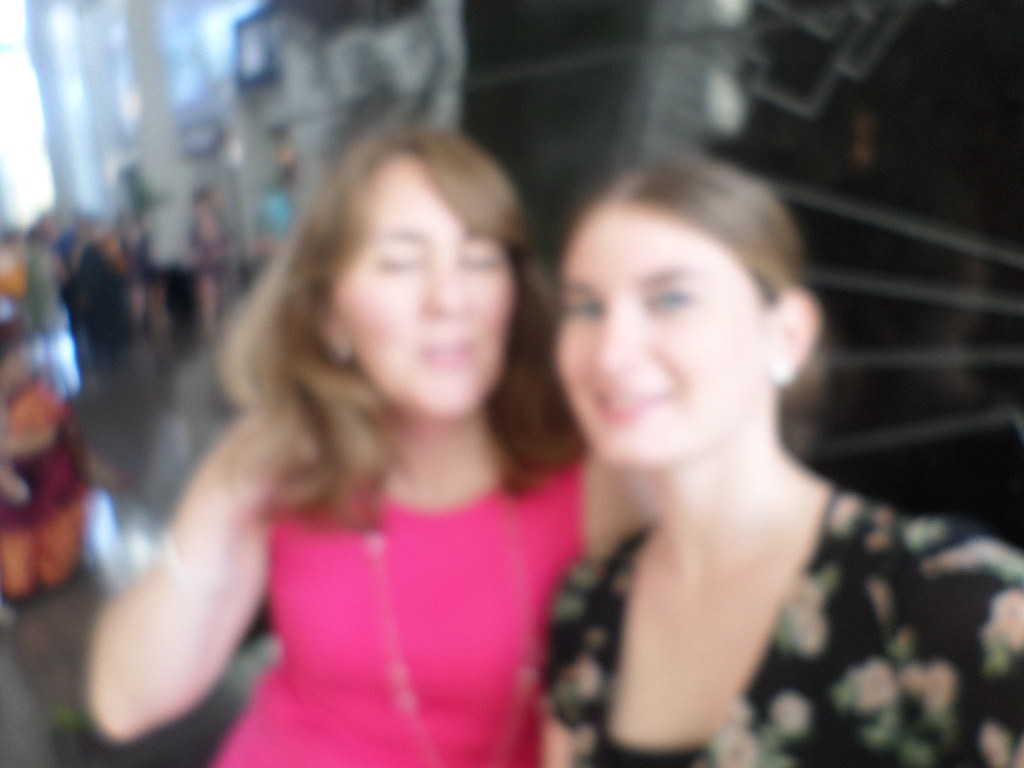In the blurry image, two white females are posing side by side, facing the camera. The woman on the right has her hair tied up and is wearing a black floral dress adorned with pink flowers that have pink centers. She has blue eyes that are faintly visible through the blur and is accessorized with small stud earrings. The woman on the left has her hair loose and short with blonde highlights. She is donning a pink top and a necklace with white beads. A strap, possibly from a pocketbook, is draped across her body from her left shoulder to her right waist. She appears to have her left hand raised, and her eyes are closed. The background features a black wall, and various indistinct objects and colors, with hints of red, orange, and brown, suggesting they might be at a shopping center, airport, or mall, along with faint silhouettes of people in the left corner of the image.